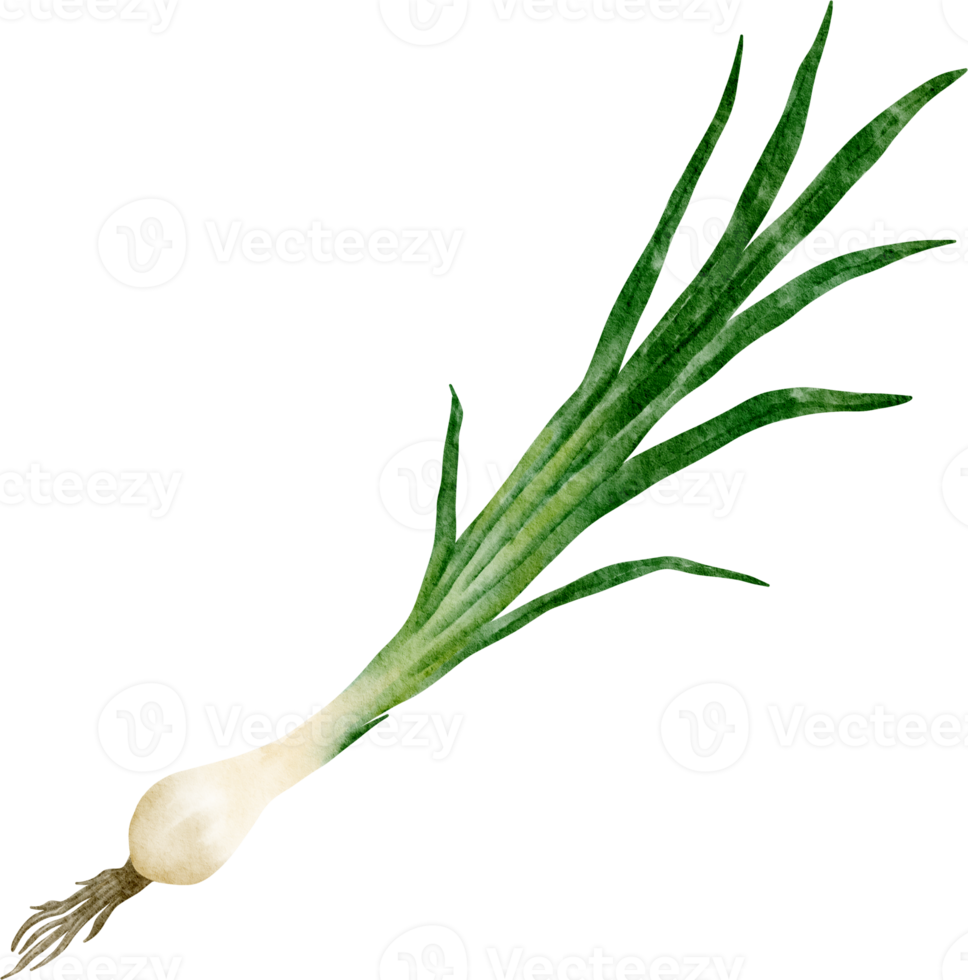This image features a detailed, high-resolution photograph of a single green onion, meticulously positioned on a stark white backdrop. The orientation of the onion is diagonal, stretching from the bottom left corner, where its short tangled roots almost touch, to the top right corner, where the green stalks narrowly miss the edge. The green onion, often mistaken for a spring onion, displays a pristine white bulb at its base, gradually transitioning into an array of light to dark green leaves toward the top. 

Overlaying the entire image is a semi-transparent watermark reading "Vecti," accompanied by a stylized "V" symbol within a circle, recurring multiple times, including across the onion itself. This watermark, though present, is designed to be unobtrusive. The seamless blend of color gradients—from tan and white at the base to varying shades of green—suggests that the image may have been digitally enhanced or created, adding to its almost animated appearance. The edges of the onion reveal a subtle cutout effect, reinforcing the notion that it may have been extracted and placed onto the white background for a clean, isolated view.